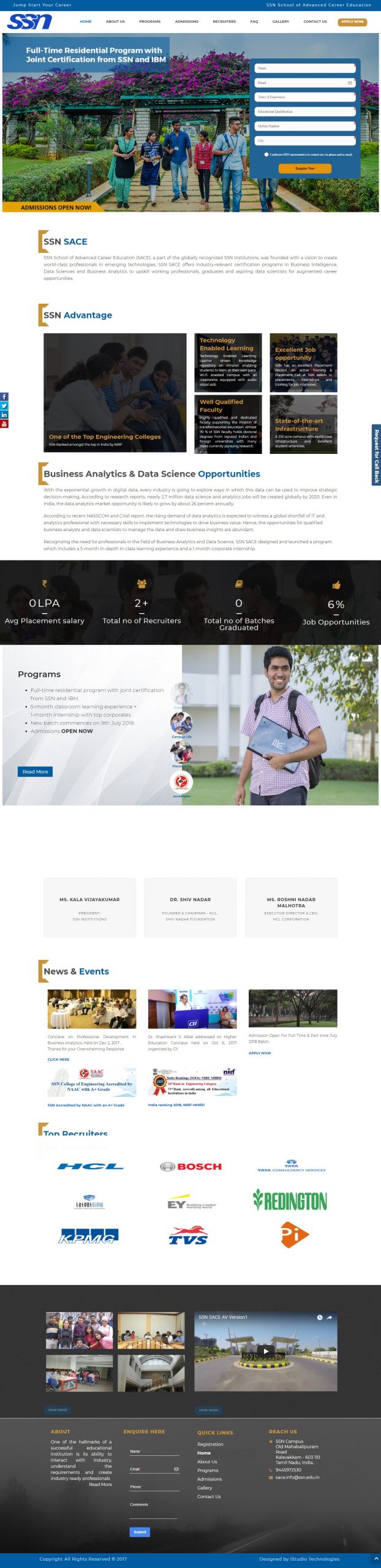The website features a clean layout with a slightly challenging readability. On the left-hand side, the acronym "SSN" is prominently displayed in blue. The homepage highlights a "Full-Time Residential Program" that offers a joint certification from SSN and IBM. The central image on the page showcases a picturesque garden scene with lush bushes, green grass, blooming flowers, and six people walking. Despite some obstruction by a pop-up asking for user information, five individuals are clearly visible, while only the legs of the sixth person can be seen on the right. The subsequent page features the bold uppercase heading "SSN SPACE," with some text underneath that is difficult to decipher. The page also touts the "SSN Advantage," presenting overlayed text on background images. The overall design combines textual and visual elements, although the text overlays on images and the pop-up might slightly hinder user experience.